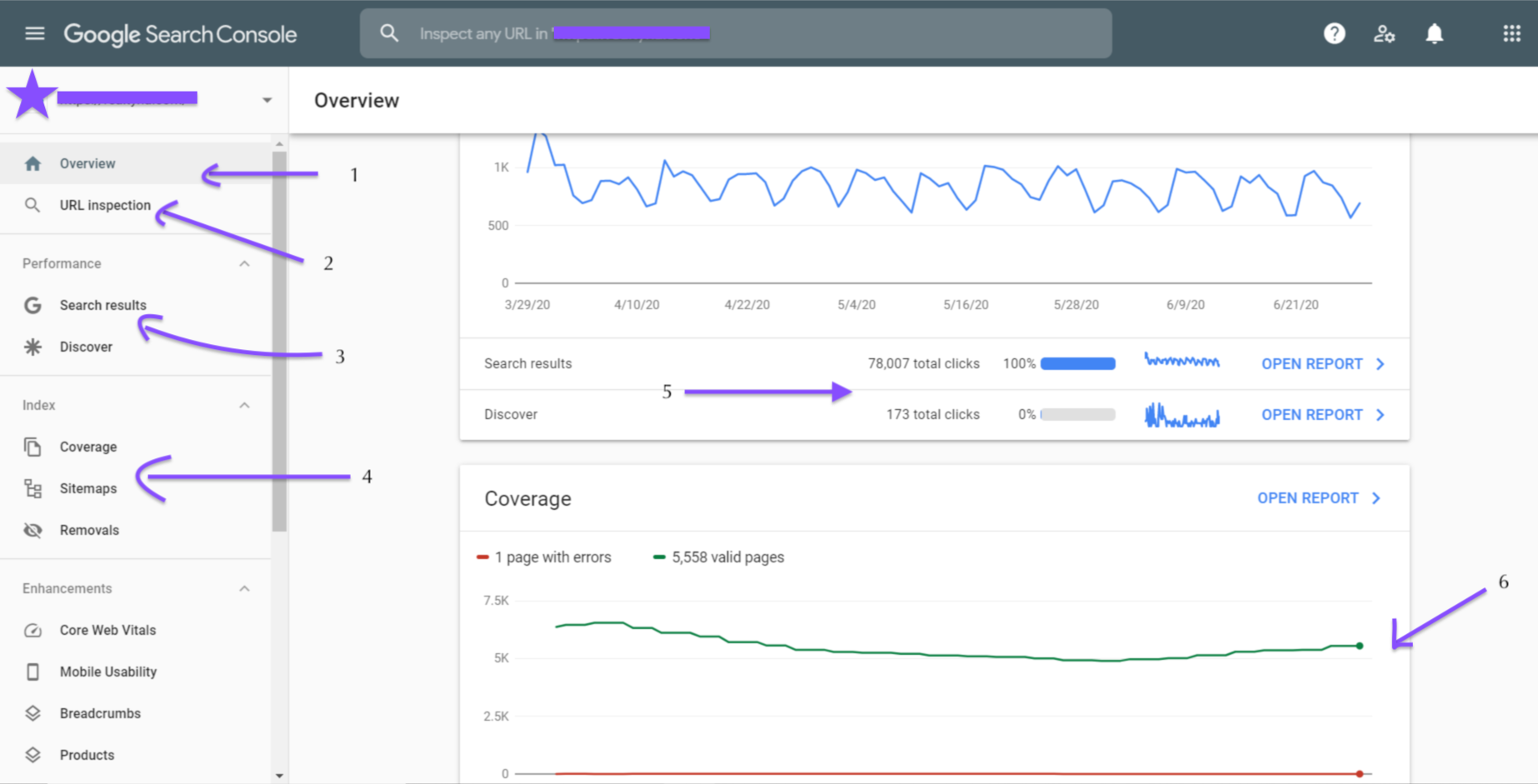Screenshot of Google Search Console webpage interface:
At the top, a grey navigation bar features a menu icon with three lines stacked, followed by the "Google Search Console" logo. Next to it, there’s a search bar with a magnifying glass icon and the text "Inspect any URL." To the right of the search bar are four icons: a help icon (question mark), a user management icon (person with a gear), a settings icon (gear), and a menu icon (grid).

Below the navigation bar is a prominent purple section with a partially obscured "Overview." Underneath, a sidebar menu starts with a home icon and "Overview" highlighted with a purple arrow marked with the number one. Below that is a magnifying glass icon labeled "URL inspection" with another purple arrow marked number two. This is followed by the "Performance" option, indicated by a Google 'G' logo and labeled "Google Search results," accompanied by a third purple arrow. The menu continues with a sun icon for "Discover," an "Index" section, a piece-of-paper icon for "Coverage," and a section for "Sitemaps," which has a purple arrow marked number four. Further down, an eye icon with a slash for "Removals," an "Enhancements" section, a cloud icon for "Core Web Vitals," a phone icon for "Mobile Usability," and a symbol with two boxes for "Breadcrumbs." The list continues with the same two-box symbol labeled "Drugs."

To the right, a data summary box displays graph visuals and key metrics: "Search results," "Discover," and "Coverage." The information includes "1 page with errors" and "5,558 valid pages."